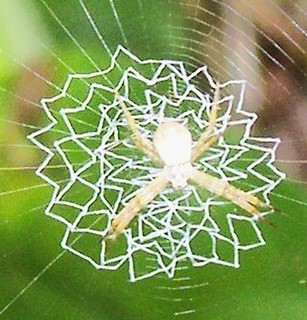This detailed image captures a fascinating spider and its intricate web. At the center of the web sits a spider with a bulbous, pill-shaped body that appears white and has a skull-like head. Its long, thick legs, which are beige with yellow and white stripes and black tips, extend in an X formation, making the spider resemble an X over the web. The web itself is a marvel, composed of very thin, nearly transparent lines forming traditional concentric circles around the periphery. However, the most striking feature is the dense, zigzag patterns in the web's center that evoke the appearance of a snowflake or woven ribbon, making it look almost surreal. The background of the image is blurred, mostly in shades of green with hints of brown and white in the upper right corner, drawing all focus to the spider and its extraordinary web.